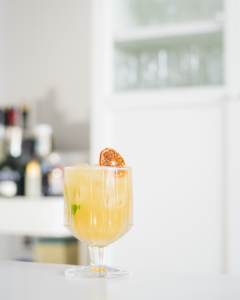The image showcases a short, stout cocktail glass, reminiscent of a half wine glass, filled with a golden-yellow mimosa. The drink appears to be based on orange juice, garnished with a mint leaf and a thin, dried slice of orange tucked inside the glass. Positioned on a white table, the drink is the central focus of the photo. In the background, which is notably blurry, there seems to be a kitchen with a white wall and a cabinet adorned with glasses. On the left side, indistinct shapes, possibly jars or liquor glasses, contribute to the scene, although they are blurred and reflective. The overall image is of low resolution, adding to the blur and indistinctness of the background elements.